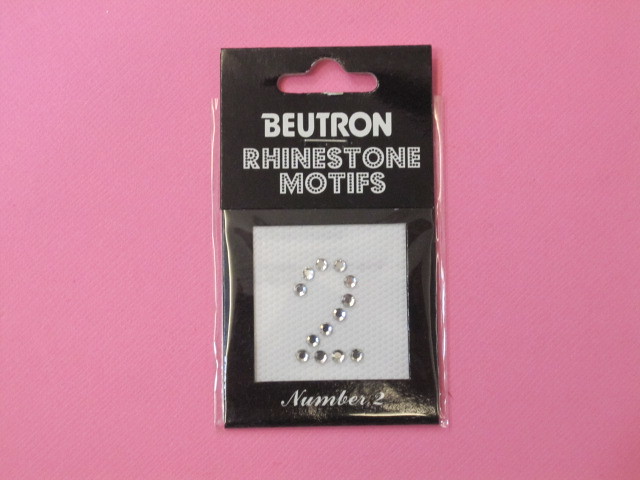The image showcases a packaged product in the center of a purplish-pink, Pepto-Bismol colored background, likely an older, low-quality photograph. The rectangular package is vertically aligned and features a black cardboard backing with a hanging cutout at the top, indicating it’s designed for display on a store rack. Centered on the black backing is the brand name, "BEUTRON," in white text, followed by "Rhinestone Motifs," also in white but with a black dotted pattern inside the text. Covering the lower part of the package is a clear plastic section through which you can see a white fabric insert. Affixed to this insert are rhinestones arranged to form the number "2." Below this, printed directly on the package in white text, is "NUMBER 2." The packaging is in the traditional style used for small jewelry items, designed to show off the clear or white-colored rhinestones prominently.